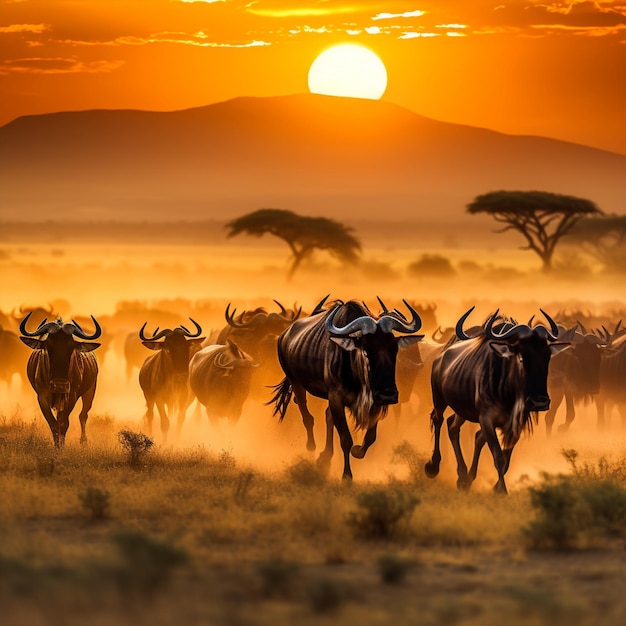The image is an illustrated depiction of a vibrant sunset on a savannah, characterized by deep orange hues that engulf both the sky and the ground. The setting sun is slightly obscured by a large mountain in the background, adding depth to the scene. The sky contains a few scattered clouds. Dominating the foreground is a large herd of wildebeests mid-stampede, with two prominently in front and clusters of others forming a dynamic, dusty trail as they seem to flee from an unseen threat. The wildebeests, identifiable by their curled horns and slight facial fur, kick up a significant amount of dust, partially obscuring those further back in the herd. The terrain features dry grass, sparse shrubs, and a few acacia trees with their characteristic flat tops, further enriching the image of the desolate yet majestic African plains.